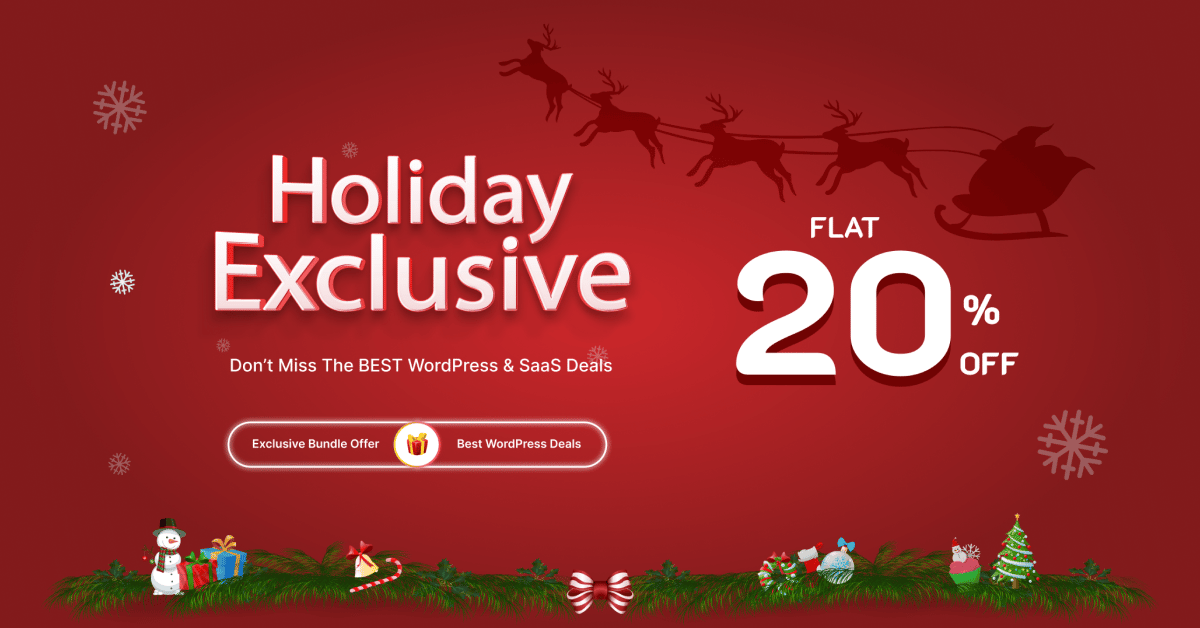Discover the ultimate holiday deal with our exclusive bundle offer! At the top, a festive banner showcases the message "Exclusive Bundle Offer: Best WordPress Deals, Flat 20% Off." A vibrant circle highlights the unbeatable promotion. Below, a meticulously rendered image displays a beautifully decorated Christmas tree adorned with red, white, and blue ornaments, including a striking wreath and a shiny ornament. Celebrate the season with the best discounts on WordPress bundles—an offer you can't afford to miss.